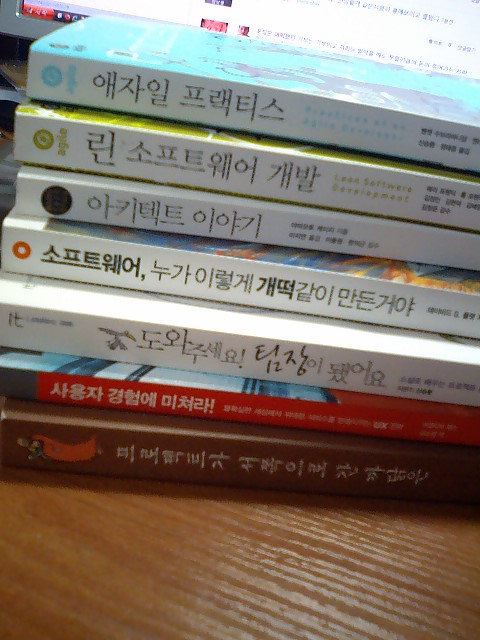The image displays a stack of seven books arranged on a brown wooden table in front of a computer screen with foreign text, likely Korean. The books are positioned with their spines visible, showing a combination of colors and distinct titles in black foreign script. Starting from the bottom, the book at the base is brown, followed by a red book with white foreign writing. The next five books are primarily white with black text. One of these white books features an orange circle on its spine, another has a black circle, the following one has a green circle, then another with a blue circle, both marked with the word "Agile." The overall setup highlights the linguistic and thematic diversity of the collection.